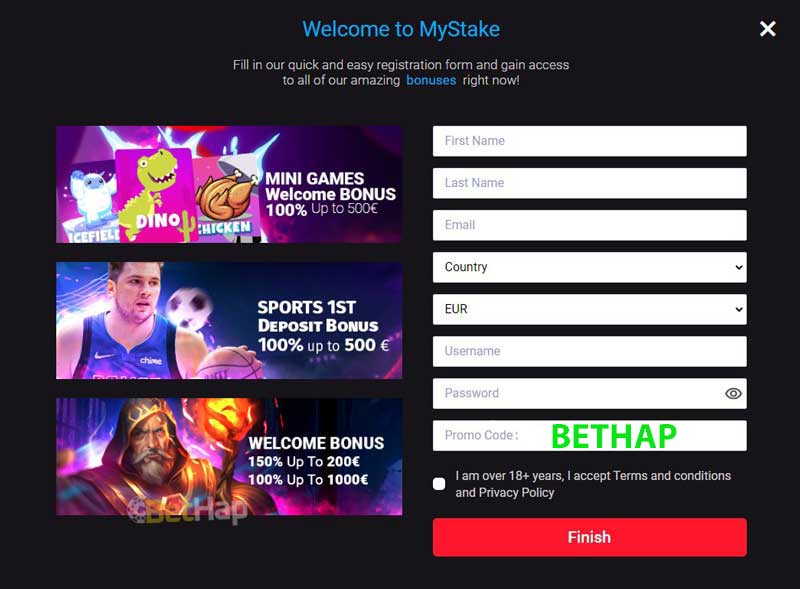The image depicts a section of a website with a sleek black background. The focal point is a square area at the center-top, featuring medium blue text that reads "WelcomeToMyStake," with the 'W,' 'M,' and 'S' capitalized. To the right of this text is a white 'X' icon.

Below the main heading, a line of text in white provides further instruction: "Fill in our quick and easy registration form and gain access to all of our amazing bonuses right now!" The word "bonuses" is highlighted in the same medium blue color as the main heading.

To the left, a vertical column features three distinct banners showcasing various promotional offers:
1. The first banner displays cartoon-style graphics associated with games, accompanied by text that reads, "Mini Games Welcome Bonus 100% up to 500 pounds."
2. The second banner has a sports theme, featuring a classic soccer player and a soccer ball, with the text, "Sports First Deposit Bonus 100% up to 500 pounds."
3. The third banner is a general promotional message reading, "Welcome Bonus 150% up to 200 pounds, 100% up to 1,000 pounds."

On the right side, there is a blank registration form with fields for "First Name," "Last Name," "Email," "Country" (with a dropdown menu), "Euro" (currency dropdown), "Username," "Password,” and "Promo Code," prefilled with "Bethapp" in lime green text. Below the form, there is a checkbox labeled "I am over 18+ years, I accept terms and conditions and privacy policy."

At the bottom, a prominent red banner with white text states, "Finish," inviting users to complete the registration process.